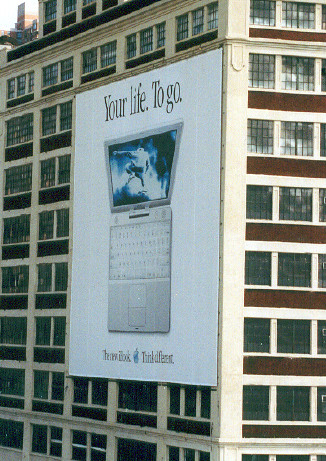This color photograph captures the corner of a very tall office or apartment building, showcasing its light cream or sandy exterior with contrasting streaks of burgundy brown and slate gray. The building features multiple stories with very large windows on each floor. The right 25% of the image reveals the front facade illuminated by sunlight, while the larger portion displays the less sunny side extending at an angle. Near the top of the building, just below a single row of windows, a massive advertisement spans over five stories. The white banner displays an Apple laptop with a silver keyboard and a bluish blurry image on its screen. Above the laptop, in bold black text, the slogan reads, "Your life to go," with smaller, unreadable black text below likely describing the product.